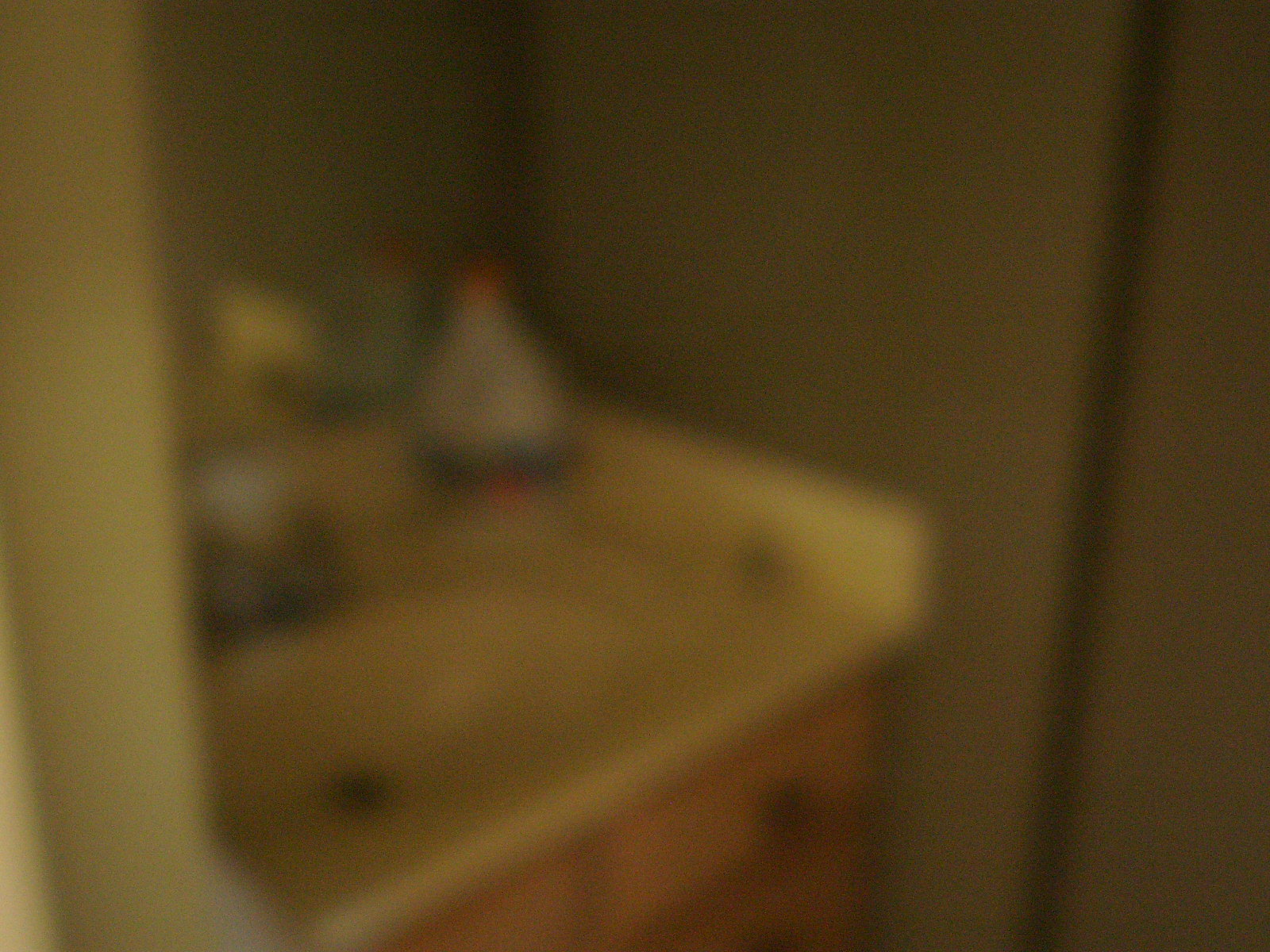This blurry, horizontally-oriented photograph appears to depict a bathroom, viewed from a first-person perspective through a doorway. The walls have a brownish or yellowish-white hue, possibly wallpapered. At the center of the image is a single, tan porcelain sink set into a light wooden cabinet with two visible drawers and additional storage below. The sink basin is aged with a yellow tint, featuring a gray faucet and a white handle. A large mirror hangs behind the sink, reflecting a prominent plastic bottle situated in the back-right corner of the basin. This bottle has a blue and orange bottom with an orange top, and although the blurry quality makes it hard to identify precisely, it is most likely a bottle of hand soap or bleach. Various bathroom items rest on the sink’s side, contributing to the cluttered impression captured in the grainy, in-motion shot. The left side of the image includes partial views of the door and doorframe.